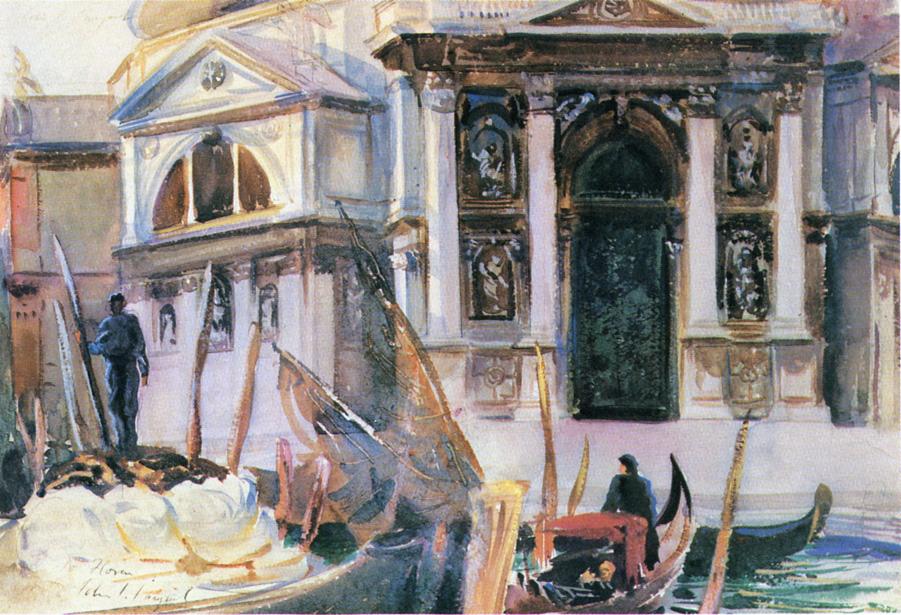The painting, rendered in an impressionistic style, depicts an imposing white or marble building that resembles a church or university. The facade of this grand structure features prominent columns and a large, tall, arched doorway that stands out due to its dark, possibly black or green, hue. Statues or reliefs are visible flanking the door and atop the triangular pinnacle of the building, lending an air of classical elegance. The building's flat top and additional statues or reliefs near a balcony enhance its grandeur. To the left, a statue stands adjacent to the building, further embellishing the scene.

The setting is adjacent to a calm, teal body of water reminiscent of Venice or Italy, where several small wooden boats congregate at a riverside dock. Among them is a larger boat carrying bundles, while another dark green gondola carries a man dressed in a long black robe and hat, suggesting he might be a person of significance. The water reflects the bright yellow light bathing the scene, though the painting itself, while bright, is not overly cheerful.

The scene captures the immaculate beauty and fine art essence of the setting with brushstrokes that evoke a watercolor feel. The combination of the serene water, detailed architecture, and classical elements creates a vivid and comprehensive portrayal of this captivating scene.